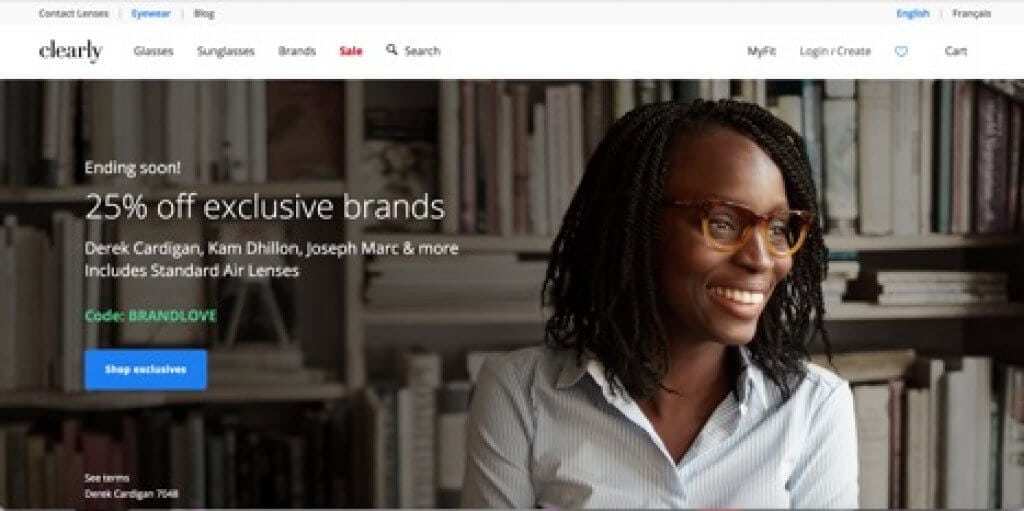The image is a detailed screenshot from a website dedicated to eyewear. At the top, a gray banner features the words "Contact Lenses," "Eyewear," and "Blog." Below this banner, the site prominently displays the brand name "Clearly" in a larger text. The navigation menu includes options for "Glasses," "Sunglasses," "Brands," and "Sale," with the word "Sale" highlighted in red. To the right, there is a magnifying glass icon accompanied by the word "Search," and links for "MyFit," "Login," "Create," along with heart and shopping cart icons.

The central part of the image showcases a graphic of a woman standing in front of a bookshelf, suggesting she is in a library. She is depicted from the chest up, wearing a pair of brown, tortoise-shell frame glasses and a white blouse with an open collar and buttons at the top. The woman has dreadlocks and is gazing slightly to her left, showing more of the right side of her face.

On the left side of the image, there is a promotional text: "Ending Soon: 25% Off Exclusive Brands. Derek Cardigan, Cam Dylan, Joseph Mark, and more include standard air lenses." This message is in green print, followed by the promotional code "BRANDLOVE." A blue tab beneath this text prompts users to "Shop Exclusives."